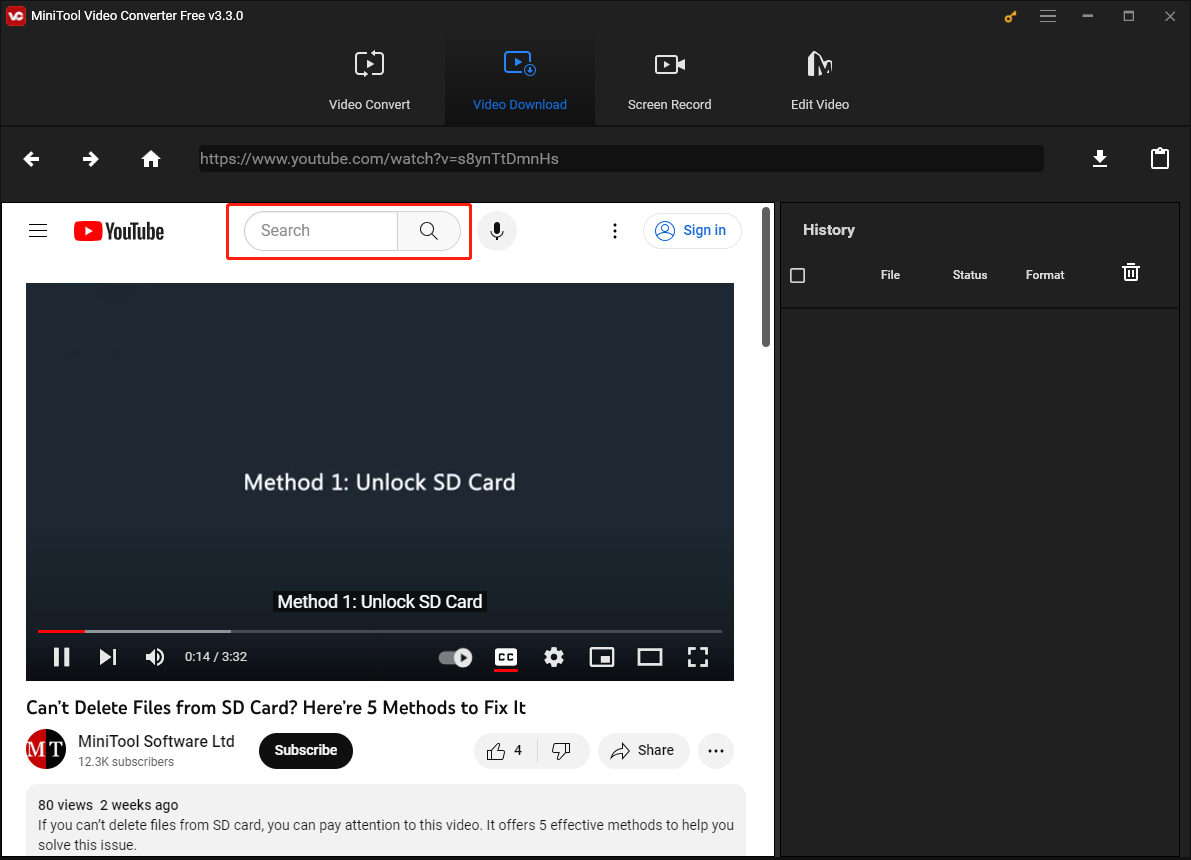The screenshot depicts a computer monitor displaying the interface of the "MiniTool Video Converter Free V3.30" software. The header section features the logo "VC MiniTool Video Converter Free V3.30" on the left, accompanied by a gold skeleton key icon, a hamburger menu, a dropdown box, and a close (X) button on the right. Below the header, there are navigation tabs labeled "Video Convert," "Video Download" (the current tab), "Screen Record," and "Edit Video."

In the toolbar below the navigation tabs, a row includes left and right-facing arrows, a home icon, and an address bar displaying "youtube.com/watch." Adjacent to this toolbar are a download arrow icon and a clipboard icon.

The main body of the page displays content from YouTube. At the top, the familiar YouTube logo, a search box outlined in red with a microphone icon, three vertical dots, and a sign-in button are visible. The video being displayed is titled "Method 1: Unlock SD card," with closed captions visible at the bottom. The video's duration is 3 minutes and 32 seconds, and the current timestamp shows 14 seconds.

Below the video, a text section reads, "Can't delete files from SD card? Here's five methods to fix it." The associated YouTube channel information includes the MT logo, "MiniTool Software LTD," 12,300 subscribers, a subscribe button, like/dislike options, a share button, and the video's view count as "80 views two weeks ago." Additional text states, "If you can't delete files from an SD card, you can pay attention to this video. It offers five effective methods to help you solve the issue."